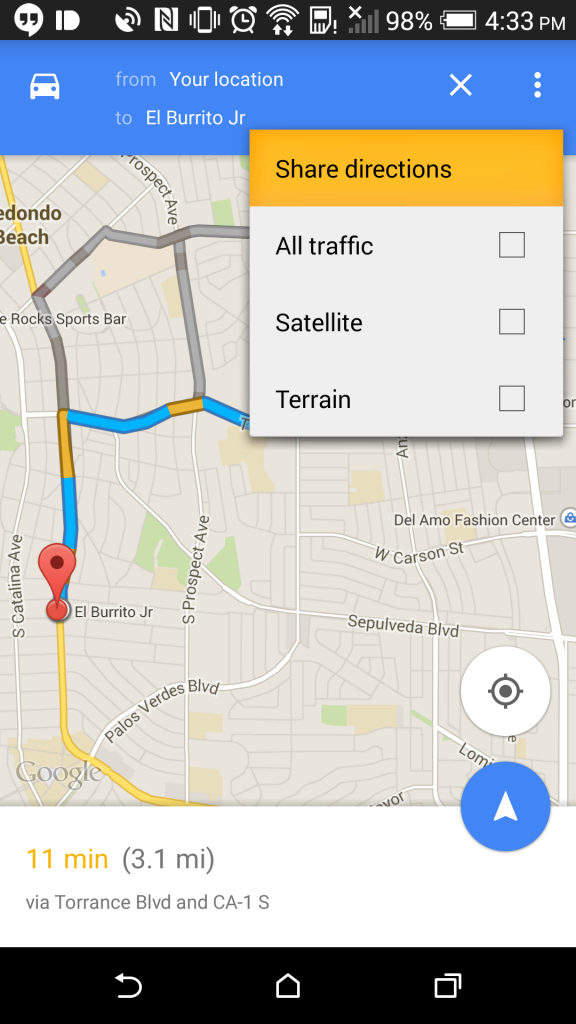The image is a screenshot of a map application displayed on a mobile device. At the top of the screen, the notification center is filled with a significant number of notifications. Below this, a blue bar features a white vehicle icon on its left, with fields for entering the starting point and destination. Positioned on the right side of this bar is a white "X."

The main portion of the screen displays a map, prominently marked by a red pin indicating the destination. A blue line outlines the route to be taken. In the upper right corner of the map, a menu box shows options for "Shared Directions," "All Traffic," "Satellite," and "Terrain," although none of these options are selected.

The route begins from "Your Location" and ends at "El Burrito Junior." The travel time is estimated to be 11 minutes, following Torrance Boulevard and CA-1S.